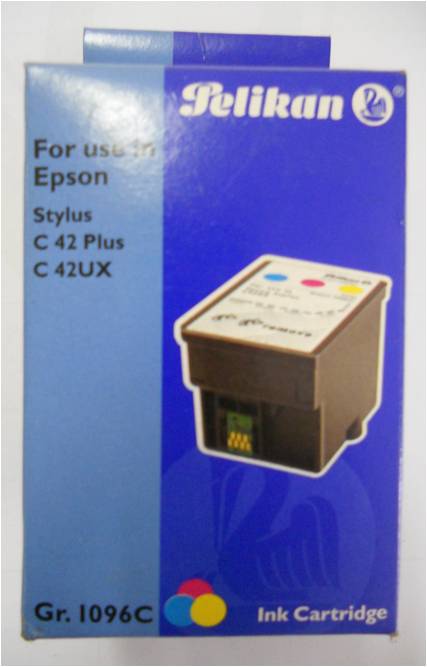The image is a portrait-mode photograph of the front of a Pelican ink cartridge box set against a light gray or light blue background. The box is predominantly divided into two sections: the left one-third is light blue, while the remaining right two-thirds is dark blue. At the top right of the dark blue section, the brand name "Pelican" appears in white font, accompanied by a pelican bird logo within a white circle. On the light blue side, black text indicates compatibility details, stating "For use in Epson Stylus C42 Plus or C42X."

Prominently displayed on the dark blue section is an image of the ink cartridge, which is gray with a white label on top, featuring three colored dots: blue, red, and yellow. These colors are repeated in three interlocking circles at the bottom of the packaging, arranged with yellow on the right, blue on the left, and red on top middle. Below the circles, the words "ink cartridge" are printed in white lettering. The serial number "GR1096C" is displayed near the bottom of the light blue section. The entire box is framed by a white background, making the packaging details stand out clearly.